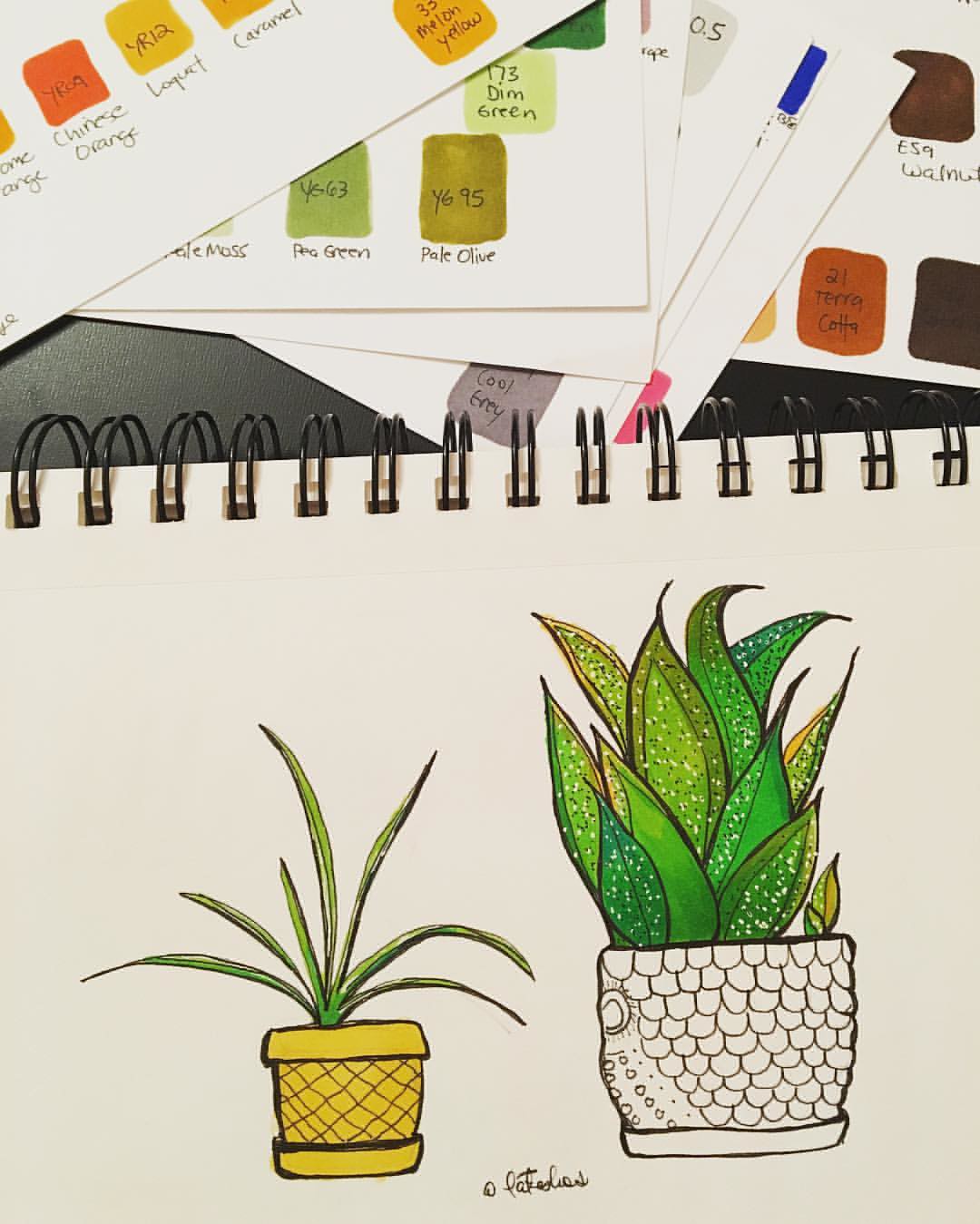This image features an open spiral-bound sketchbook with visible black metal rings at the top, holding white paper. The focus is on two detailed drawings of potted plants. The left pot is yellow with a black checked pattern resembling diamonds, containing a plant with approximately seven green leaves sprouting in various directions. The right pot is uncolored, detailed with intricate black pencil drawings resembling fish scales and an eye, possibly evoking a mermaid theme. Its plant has thick, green leaves speckled with white, numbering around ten, varying in height. An artist's signature is present between the two pots, though only partially legible, appearing to start with "Pat."

Above the sketchbook are small cards displaying watercolor swatches labeled with both names and codes, such as "Pale Olive Y695" and others like "Pea Green" and "Dim Green." The scene captures the artist's meticulous work and their color reference materials, offering a glimpse into their creative process.